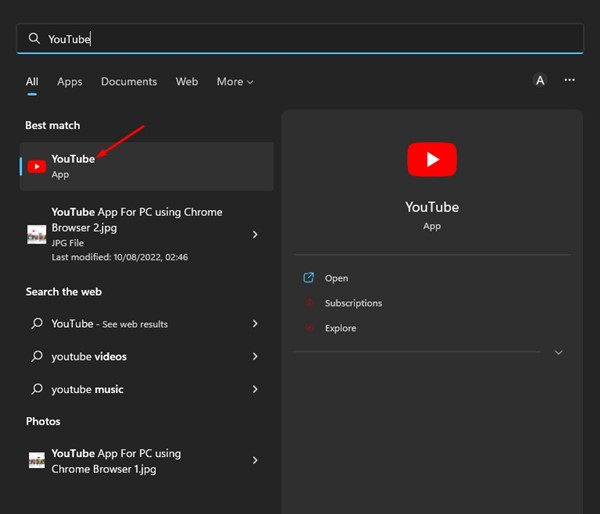The image depicts a computer screen displaying the search results for the term "YouTube" on a search page. At the top, in the search area, the word "YouTube" is being typed, accompanied by a slim blue underline. Below the search area, several categories are visible, including "All," "Apps," "Documents," "Web," and "More." The first search suggestion under "Best match" is "YouTube," and from this point, a short red arrow, approximately an inch long, points diagonally from the top-right to the bottom-left of the screen.

Further down, the search results continue with "YouTube app for PC using Chrome." The next section offers options to "Search the web" with listings like "YouTube," "See web results," "YouTube videos," and "YouTube music." Continuing down the results list, the user can also find "Photos," and an image file titled "YouTube app for PC using Chrome browser 1.jpg."

Finally, on the right-hand side of the screen, there are additional options related to "YouTube," including buttons for "Open," "Subscriptions," and "Explore."